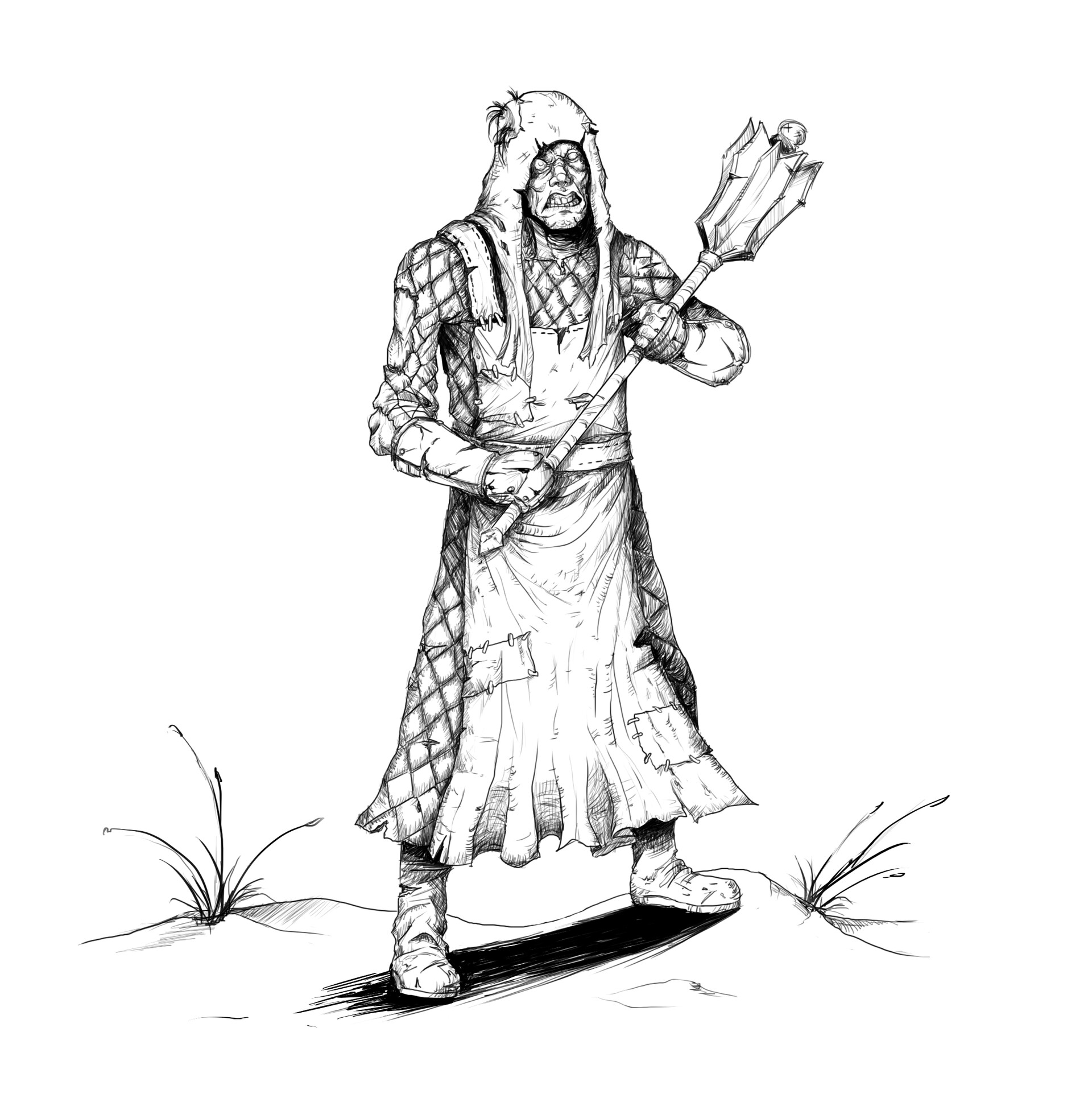The image is a detailed black and white drawing of a fictional, humanoid creature with a grotesque, misshapen face that showcases all its teeth. The creature is donning a canvas-like hat and is dressed in a patchwork ensemble resembling a battle-worn armor or suit. The outfit includes an apron-like dress with a diamond-shaped, possibly scaly pattern that extends down its body, paired with canvas boots. The creature appears intimidating, holding a large, pointy mace with a golden tip, which takes up much of its upper body. It exudes a menacing aura, standing in a shadow cast on an uneven, sandy ground with scattered plants. The entire scene exudes a sense of readiness for combat, emphasizing the creature's fierce demeanor.